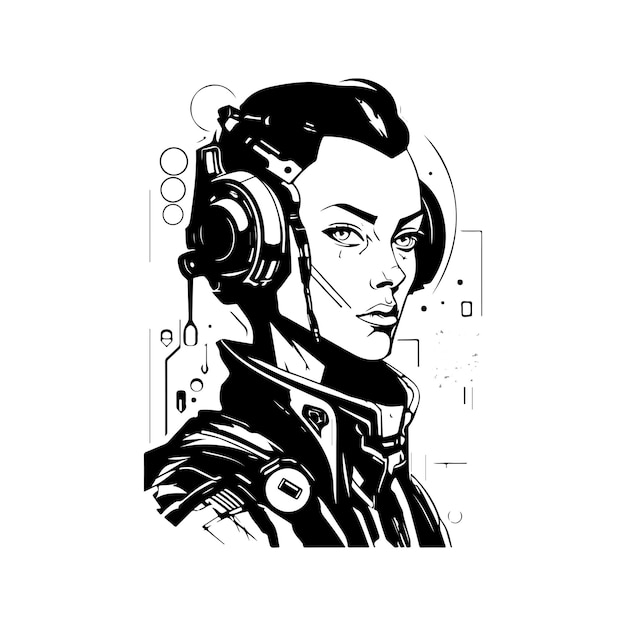This digital black and white hand-drawn image showcases a futuristic woman with short, dark hair tied back. She is adorned with a high-collared, structured jacket that suggests a solid, possibly non-fabric material, fitting the sci-fi theme. The woman wears a headset with a microphone extending to her mouth, and an additional antenna-like feature on the headphones. A glass shield covers her eyes, giving her an astronaut or flight controller appearance. Behind her, the background consists of geometric shapes, including circles and squares, potentially representing computer circuitry or equipment. The overall composition is rendered entirely in black and white, with stark contrasts highlighting the sleek, modern design.